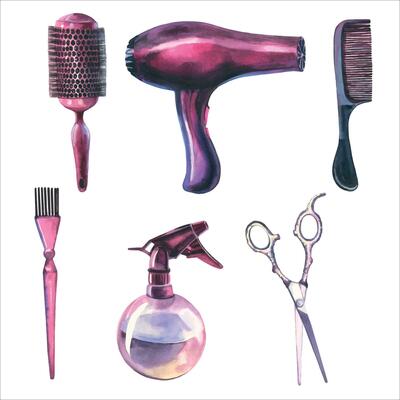The image is a square with a thin gray border set against a white background, featuring various hairstyling tools meticulously arranged. In the top row, starting from the left, there is a round brush with a purplish-pink handle and black bristles all around it. Positioned in the upper center is a purplish-black hairdryer angled to the right, and in the upper right corner, there's a black comb also pointing right. In the bottom row, beginning from the left, there appears to be a pink-handled brush, possibly for eyebrows, with long black bristles. The lower center hosts a purple spray bottle with a round base and a darker purple mister top, containing some liquid. Finally, in the lower right corner, there's a slightly open pair of silver scissors. All the objects are stylized drawings, collectively evoking a hair salon setting.